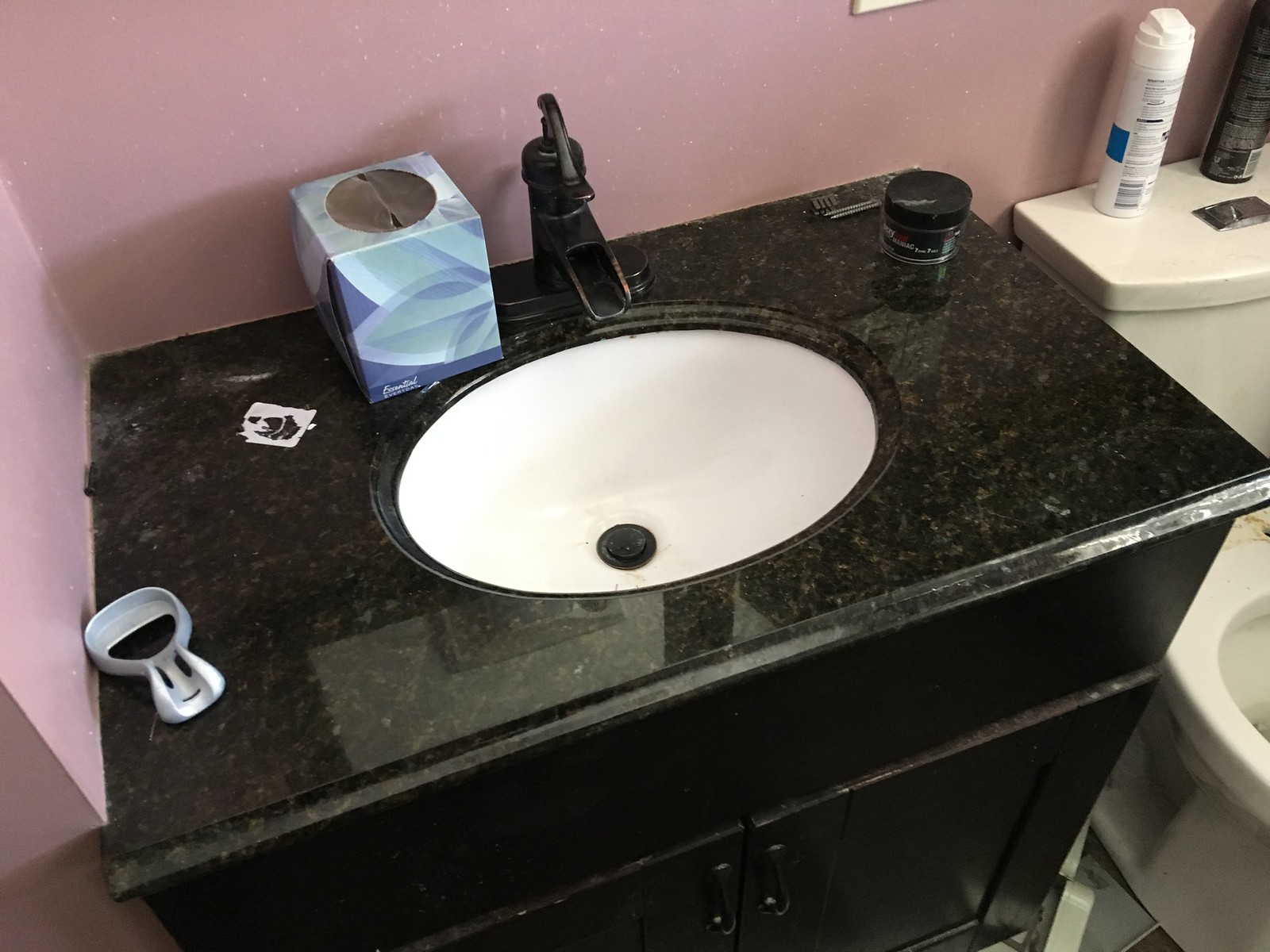The image depicts a somewhat low-resolution photograph of a bathroom corner. Dominating the scene is a black countertop nestled in the corner with a sink centrally positioned. On the countertop, there is an empty tissue box and some scattered remnants that might be residues from personal care products. In the bottom left corner of the counter, there is a holder potentially for a hairbrush or toothbrush. The upper right corner is cluttered with a few screws and a small, indistinct pot with an unreadable label due to the image's blurriness. To the far right of the frame, an open toilet is visible, with a flush button on its tank lid. Two unidentified cans are placed on the toilet’s tank, their labels turned away from the camera. The bathroom walls are painted in a dusty pink or mauve shade, adding a muted warmth to the space. Below the counter, a series of cupboards provide additional storage.